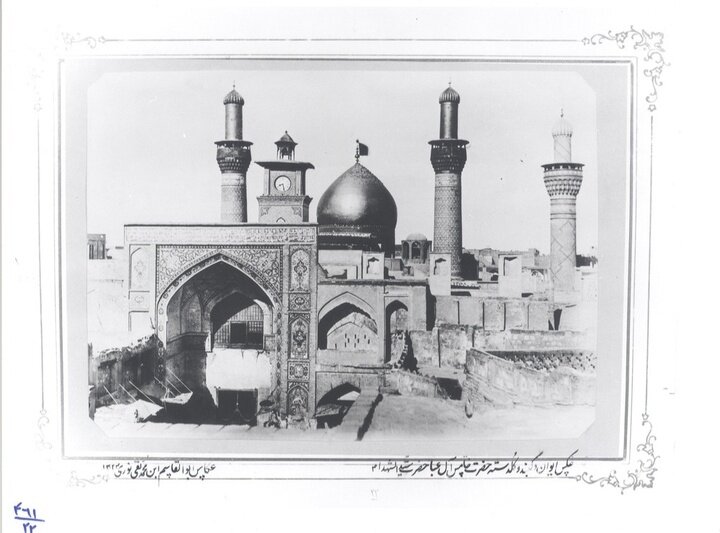The image depicts a detailed black and white drawing of a mosque with a prominent dome situated toward the middle top of the illustration. The scene is densely filled with an array of towers and turrets rising from the cluster of buildings that dominate the lower half of the image. Among these structures, an ornately decorated archway stands out on the left-hand side, hinting at an entrance made possibly of stone, featuring intricate engravings and a grand arch.

In the center of the image, past the primary arch, another arched entrance can be seen, leading the eye to the large dome behind it. This central dome, appearing to be golden in the description, is topped with a flying flag. Adjacent to the dome is a slender pole topped with a structure resembling a lighthouse, possibly indicative of a shrine. Further to the right is a smaller, similar structure with a white top reminiscent of a candle on a candlestick. On the left side of the dome sits a clock tower with a visible clock, and to its left, another shrine, similar in appearance to a candle on a candlestick, stands.

The background fades into a pale gray sky, providing a stark contrast to the intricate foreground. The image is bordered with decorative swirly lines in the corners, and at the bottom, there is some writing in a foreign language, not in English. This text is positioned on both the left and right sides of the lower border.